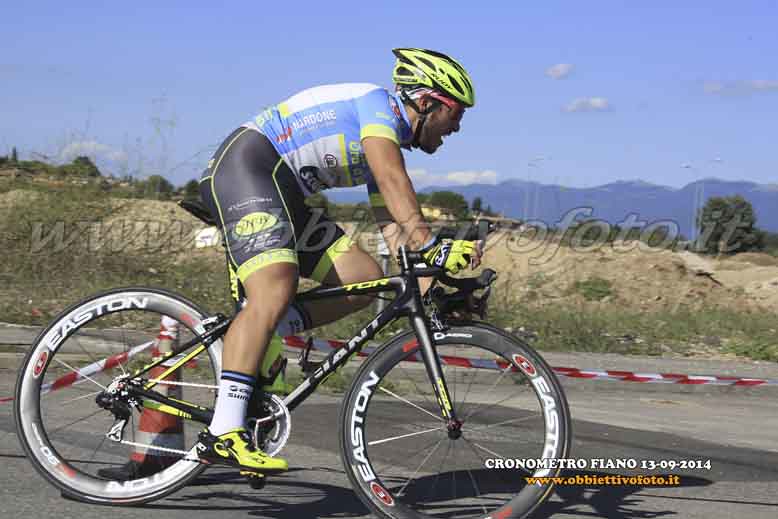The image captures an outdoor scene during the daytime, featuring a cyclist in competitive attire, racing down an open road. The cyclist wears a fluorescent green bike helmet, a blue and white jersey with white text spelling out "A-R-D-O-N-E," and black spandex shorts with yellow accents and the letters "N-B" on them. He also sports yellow and black bicycle gloves, white socks, and black shoes that are predominantly green at the front. He is riding a black bicycle with "Easton" written on the tires and "Giant" on the main bar. The cyclist's mouth is open, indicating a competitive effort.

In the background, a scenic landscape unfolds with a series of mountains layered in the distance. The mountains display hues of blue and brown, interspersed with grass and light brush. The sky above is a vibrant blue, dotted with white clouds. The scene includes a mix of grass, dirt, asphalt road, and pavement. An orange traffic cone with white stripes is visible near the cyclist's back tire.

The bottom right-hand corner of the image displays the text "Chronometrofiano 13-09-2014 www.obbietto.it." The overall atmosphere is dynamic, showcasing the cyclist in motion against a beautifully detailed natural backdrop.